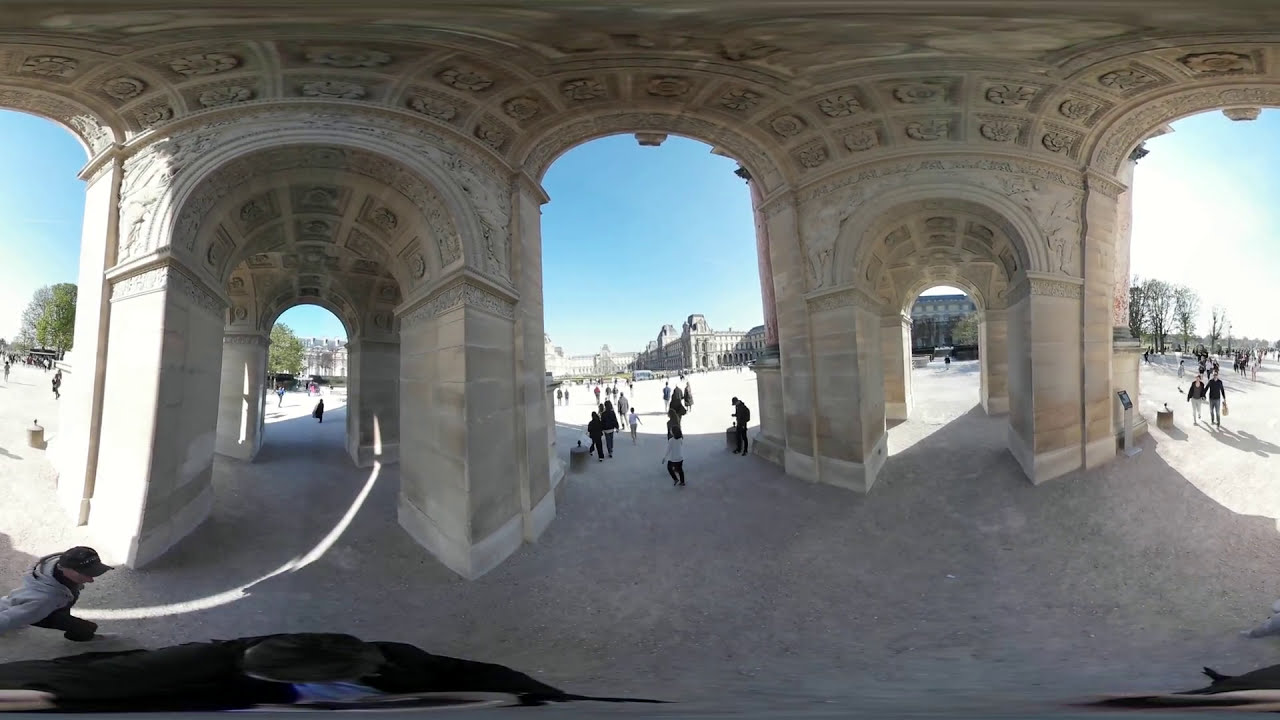The photograph captures a detailed, panoramic view of a vast stone archway structure reminiscent of the Arch of Triumph. This magnificent edifice, supported by four massive stone pillars, forms a cylindrical column shape with two large arches on the left and right and a central archway connecting them, allowing passage through the middle. The stone of the archway is gray, casting significant shadows, contrasting with the bright, blinding sunlight outside. The intricately carved ceiling adds to the ornate charm of the structure. A small crowd of people, appearing dwarfed by the grand arches, can be seen congregating around and walking through the archways, many taking photographs. The ground beneath the arch is a bare, gray surface, while the surroundings outside the archways display lush trees on both sides and a distant view of old, elaborate buildings under a clear, blue sky. It is a sunny day with no clouds, indicative of spring or early autumn, suggested by the cool-weather attire of the people, including a man in a hat and hoodie beginning to pass underneath the arch.